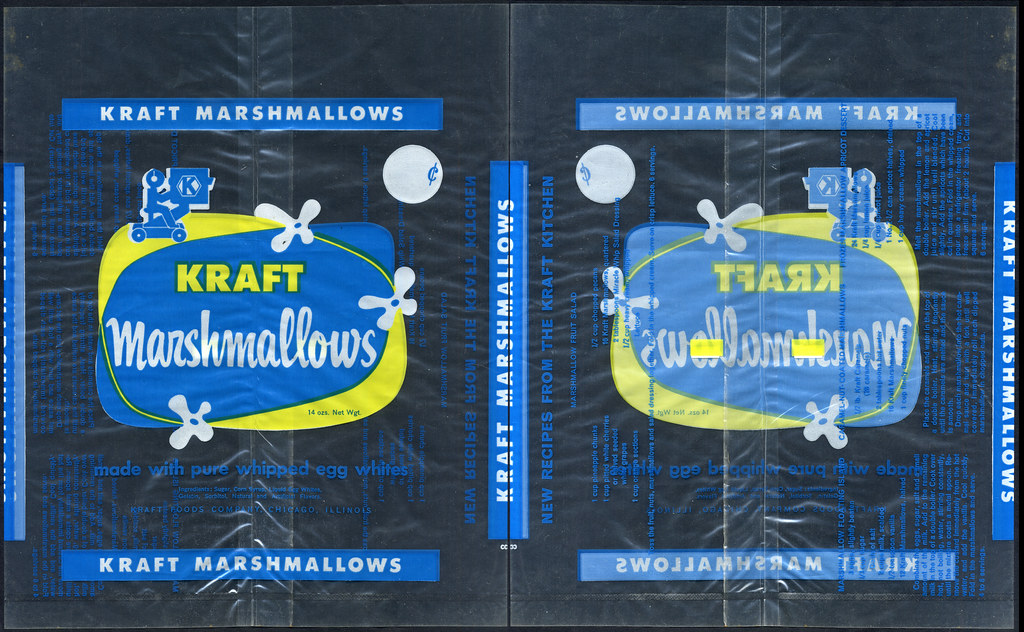The image showcases a double view of a Kraft marshmallows wrapper against a black background. The wrapper is duplicated, showing both the front and reverse sides. The top and bottom of the wrapper feature blue boxes with "KRAFT MARSHMALLOWS" written in bold, white, capital letters. The middle section of the wrapper has a patterned blue background with small text that reads, "New recipes from the Kraft kitchen," followed by more very tiny, unreadable text. Central to the forward-facing wrapper, there's an overlapping blue and yellow icon prominently displaying the word "KRAFT" in bold yellow capital letters. Below it, "marshmallows" is scripted in white cursive font. Three white flowers, reminiscent of 1960s design, and an illustration of a person on a wheeled platform holding a box marked with a "K" are also present, adding to the retro appeal of the packaging design.